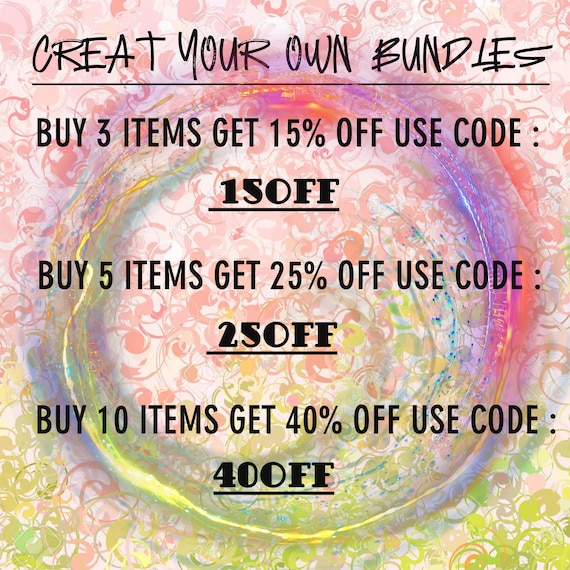This colorful advertisement features a vibrant background transitioning from predominant pinks at the top to greenish yellows at the bottom, with a central circular design surrounded by a blended gradient and an outer lip. The floral and spiraled motifs add a lively and decorative touch to the illustration. In bold black text, the main offer reads "Create your own bundles," though "Create" is misspelled and missing the "E" at the end. Promotional details include: "Buy 3 items, get 15% off, use code 15OFF," "Buy 5 items, get 25% off, use code 25OFF," and "Buy 10 items, get 40% off, use code 40OFF." No people, animals, or motorized vehicles are depicted in the advertisement.